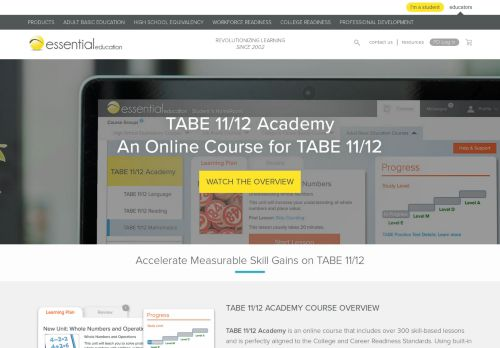**Caption:**

This image is a screenshot from the Essential Education website, identified by its yellow icon and branding where "essential" and "education" are both in lowercase letters. At the top of the page, there is a dark gray navigation bar with options listed from left to right: "Products," "Adult Basic Education," "High School Equivalency," "Workforce Resources," "College," and another option starting with "Professional" that is slightly blurred. 

The center of the image prominently features text in the largest font, reading "TABE 11/12 Academy, an online course for TABE 11-12." The primary visual element shows the upper portion of a laptop displaying the mentioned webpage. Central to the image is a square overlay with a play button, labeled "Watch the Overview," indicating that a video overview is available to view.